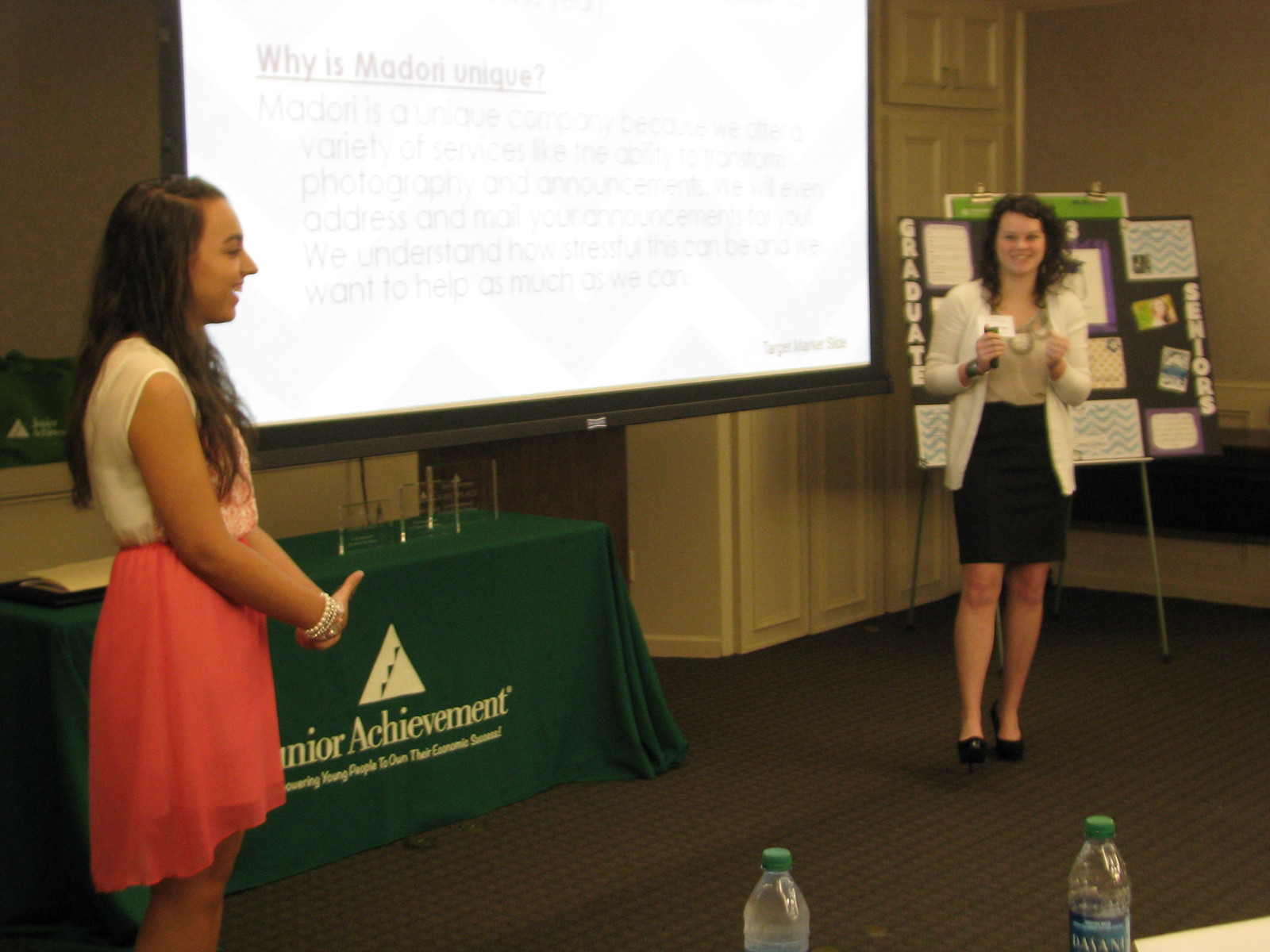In a carpeted room reminiscent of a hotel setting, two women are delivering a presentation in front of a large white screen with the title "Why is Madonna Unique?" between them. Flanking the screen are tables with green tablecloths emblazoned with the Junior Achievement logo. The woman on the left wears a white blouse paired with an orange-colored skirt and many bracelets, her long dark hair cascading down as she smiles. The woman on the right dons a white blazer over a beige shirt with oval details, a black skirt, and black heels. She also has long brown hair and is smiling. Behind the woman on the right, there is an easel displaying informational documents, with words like "graduate" and "seniors" visible on either side. Bottles of water are placed in the foreground, presumably for the audience, though they are not visible. The room also features brown walls and cabinetry, completing the professional yet inviting atmosphere.